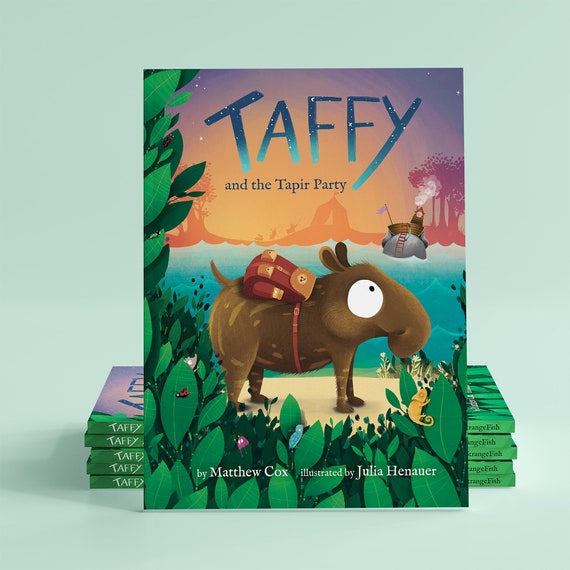This is a detailed photograph of the cover of a children's book titled "Taffy and the Taper Party." The cover prominently features big text displaying the title, with "By Matthew Cox, illustrated by Julia Hanyuar" written in smaller white text at the bottom. The illustrated cover shows a cartoonish taper, resembling a boar with a curled snout, standing on what appears to be a sandy area with the ocean or a lake behind it. This taper, named Taffy, has a cheerful expression and is wearing a leather backpack fastened around its middle. The background of the cover illustration includes a distant tent near the water, which is almost washed out due to its distance. 

In the foreground, the scene is vibrant with forest leaves arranged along the left and bottom borders, creating an L-shaped frame. Among the leaves are various critters such as an old-world chameleon, a blue beetle, a ladybug, and other barely noticeable insects like moths and butterflies. The book itself is standing upright on a mint green table or background, with five more copies stacked behind it, their spines facing outward towards the viewer. The overall illustration style is whimsical and colorful, typical of children's literature, making Taffy's adventure come to life for young readers.